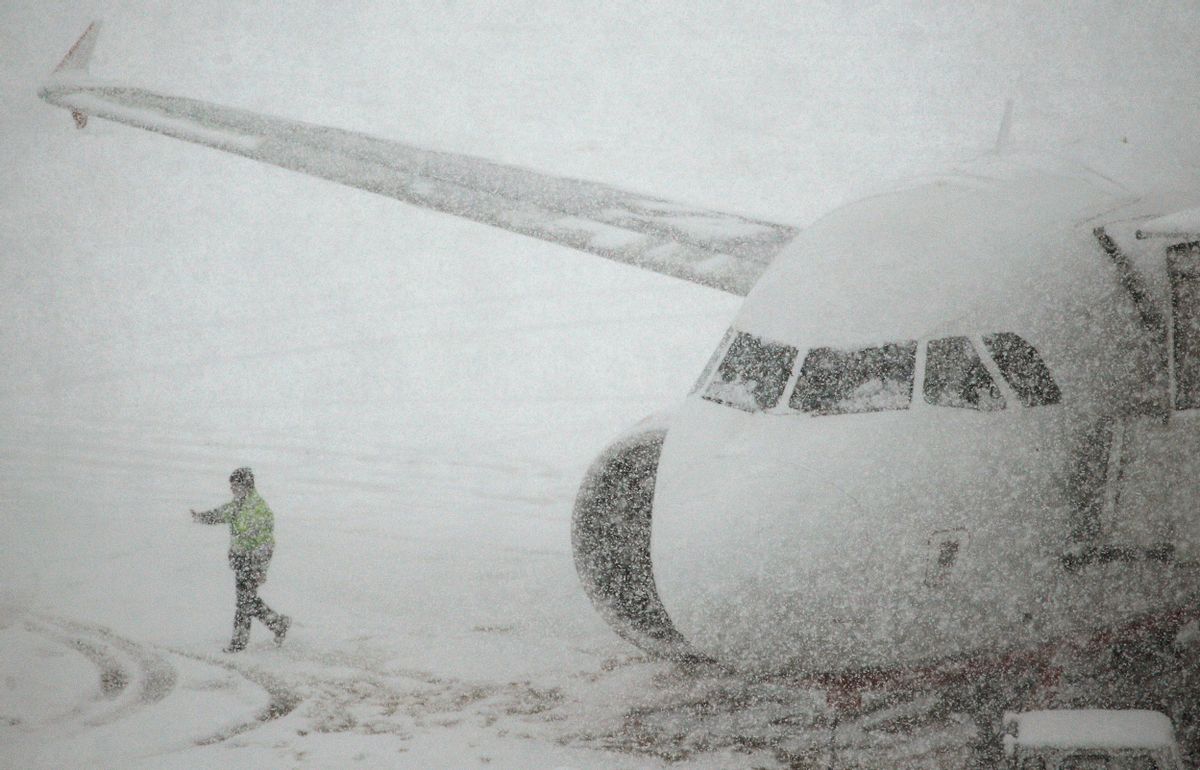A snowy, black-and-white scene reveals the front of an airplane, possibly an Airbus, with just the cockpit, right wing, and engine visible amid the snowstorm. The aircraft's nose and wing are blanketed in snow, contributing to the image's overall fuzzy appearance. The cockpit has four visible windows, while the wing features an interesting winglet design. Nearby, a person in dark pants, a dark hat, and a slightly green jacket with a reflective safety vest is walking away from the plane towards the right, leaving tire tracks in the snow. Another individual, possibly directing the plane, stands to the left in a yellow coat. To the right, part of what appears to be a door or boarding area is slightly visible through the snowy veil. The persistent snowfall washes out most colors, casting the entire scene in shades of white, black, and gray.